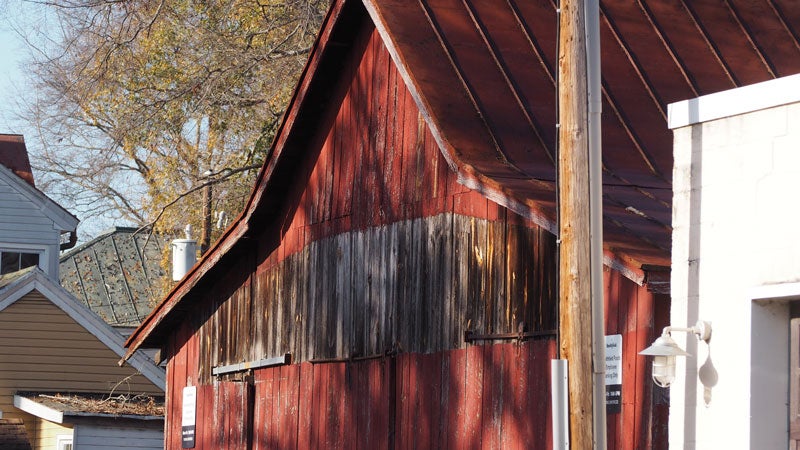This photograph captures a street scene dominated by a large red wooden building, resembling a barn, at the center. The image, taken from a close angle, starts midway up the buildings, giving it a likely residential feel, although no path or road is visible. To the right stands a small white-painted brick building with a door adorned by a sconce. The central red barn-like structure features mostly painted red sides, but just below the roof, the unpainted, age-worn wood peeks through in a grayish-brown hue. On either side of this building, small black-and-white signs are visible. Flanking the dominant red structure on the left are more residential properties with a sandy brown and grayish-whitish color palette, also wooden in construction. A telephone pole or power line pole can be seen in the foreground. The background reveals a tree with thin, spindly leaves, hinting at the fall season as the trees exhibit a yellowish-brown color and are missing many leaves. A glimmer of blue sky can also be seen in the backdrop.